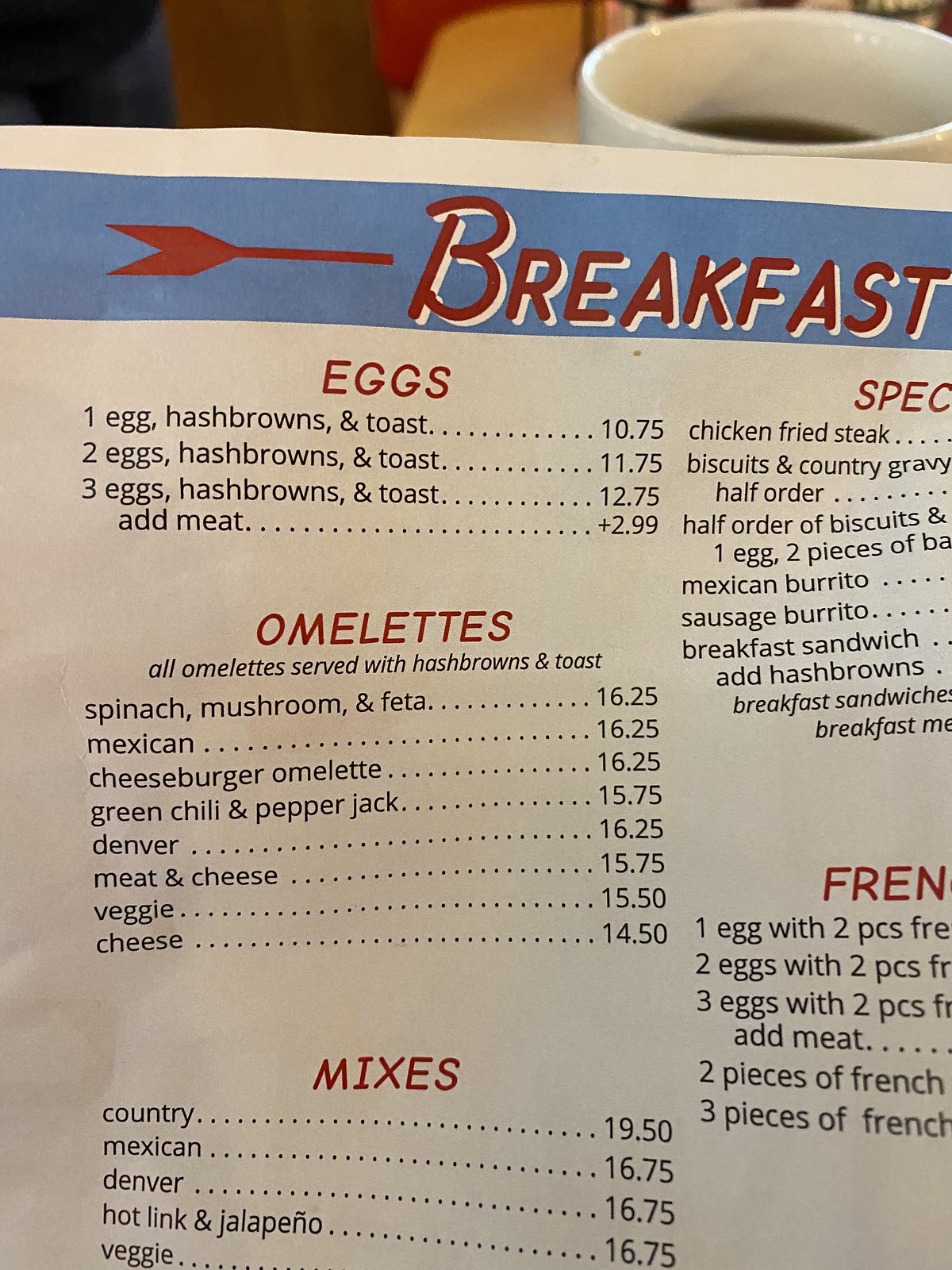The photograph prominently features a menu taking up most of the image, with a glimpse of a white coffee cup filled with black coffee at the top, resting on the edge of a wooden table. The menu is printed on a white page with a black horizontal rectangle at the top, featuring the word "Breakfast" in dark red font, accented by a white drop shadow. The right edge of the menu is cut off by the photograph’s margin.

Below the "Breakfast" header, the word "Eggs" is highlighted in red, followed by a list of three different egg dishes. The menu continues with the heading "Omelettes" in red, under which eight types of omelettes along with their prices are listed. At the bottom of the image, the word "Mixes" appears in red, indicating a category with five listed items, though more might be present since the bottom is obscured by the photo's edge.

On the right side of the menu, the partially visible word "Specials" is seen in red, along with a list detailing the restaurant's special offerings. Further down, the red letters "F-R-E-N" are visible, likely indicating a "French" category, under which five variations of French toast are listed.